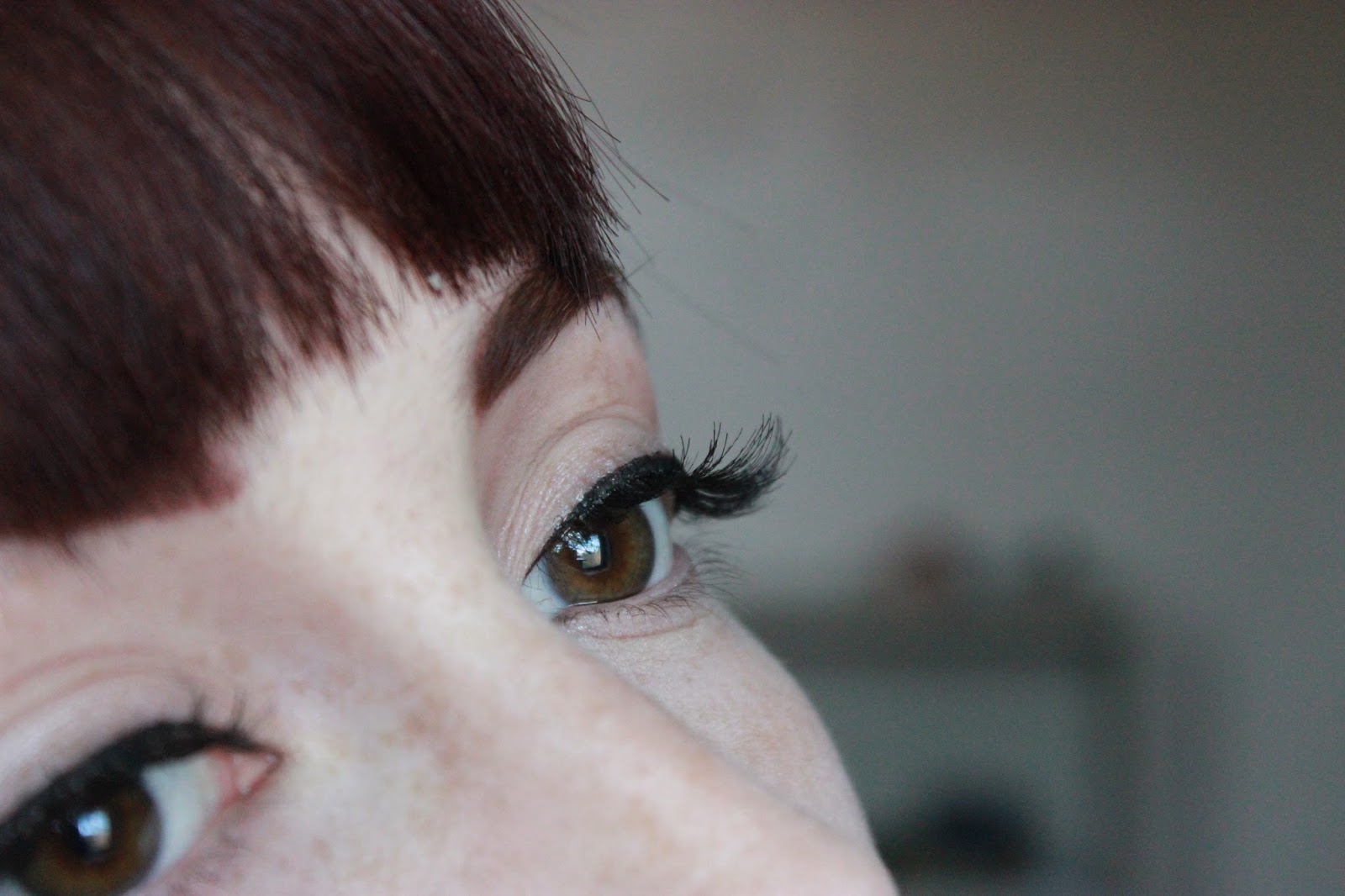In this highly detailed close-up image, a young woman is captured in a side profile, occupying the left half of the frame. Her appearance strikingly resembles Audrey Hepburn, although she is not. The focus narrows in on her expressive brown eyes, part of her nose, and her forehead, framed by light to medium brown hair and brown eyebrows. She has long, black eyelashes accentuated with black eyeliner, giving her eyes a wistful, perhaps mildly yearning expression as she gazes upward toward the right side of the image.

The background, occupying the right half, is a blurry, indistinguishable scene that vaguely suggests an indoor setting, potentially a bedroom with hints of shelving units. The image's color palette includes shades of brown, peach, black, and pink. Despite the presence of the photographer, the composition conveys a sense of solitude and deep contemplation, as if the woman is pensively reflecting on life's intricacies. Through the reflection in her eyes, a glimpse of a window or an electronic device is visible, heightening the intimate, introspective mood of the photograph.